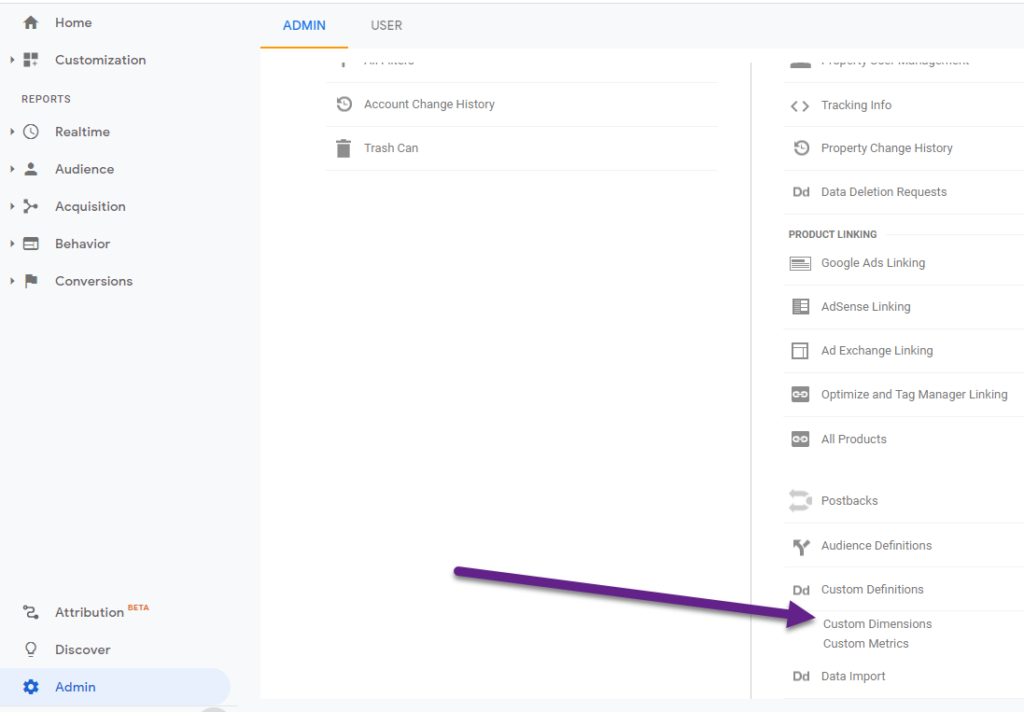The image depicts a detailed web page interface, primarily with a light gray background at the top. At the very top, there is text that reads "Home, Administration, User," where "Administration" is highlighted in blue and underlined in gold. Below the "Home" section, there is a vertical navigation column listing the following sections: "Customization," "Reports," "Real-Time," "Audience," "Acquisition," "Behavior," and "Conversions." Below this cluster, a larger gap leads to additional sections titled "Attribution," "Discover," and again "Administration," which is also highlighted in blue, matching the top highlight.

Under "User," some text is partially cut off, but visible items include "Account Change History" and "Trash Can." The midsection of the page features a large, long purple arrow running from the center to the right diagonally, labeled "Custom Dimensions, Custom Metrics."

On the right side of the interface against a white background, some text is cut off. Subsequently, the following sections are visible: "Tracking Info," "Property Change History," "Data Deletion Requests," and under "Product Linking," there are options for "Google Ads Linking," "AdSense Linking," "Ad Exchange Linking," "Optimize," "Tag Manager Linking," and "All Products." Additional sections include "Postbacks," "Audience Definitions," "Custom Definitions," with "Custom Dimensions" and "Custom Metrics" indicated again where the purple arrow points. The final label in view is "Data Imports."